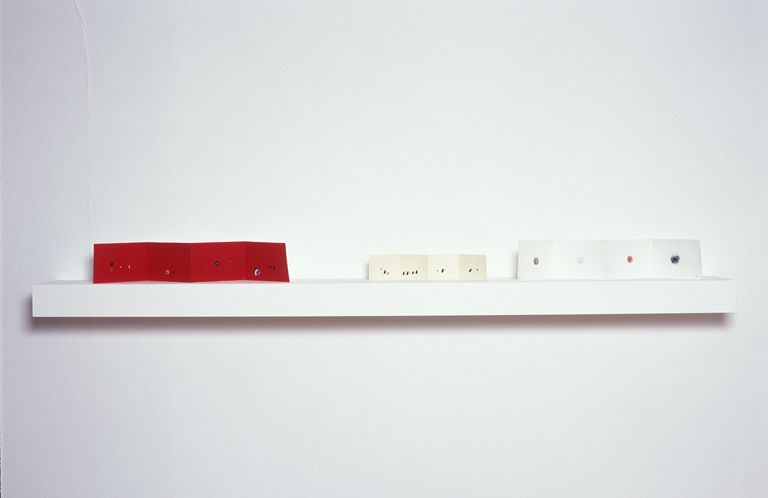The photograph captures an art display mounted on a white wall that gradually shades to gray at the edges. A thin vertical seam is visible in the top left corner. Centrally positioned just below the middle of the image, a horizontal, thin white shelf juts out from the wall, casting a dark gray shadow beneath it. On this shelf, three intricately folded rectangular papers are arranged. To the left, a red piece of paper, folded three times, features tiny polka dots and designs. In the middle, a smaller beige piece of paper, also folded three times, has delicate, scattered specks. The right side holds a white piece of paper with three folds, each displaying a single speck. These papers rest upright against the wall, contributing to the minimalist and abstract aesthetic of the composition.